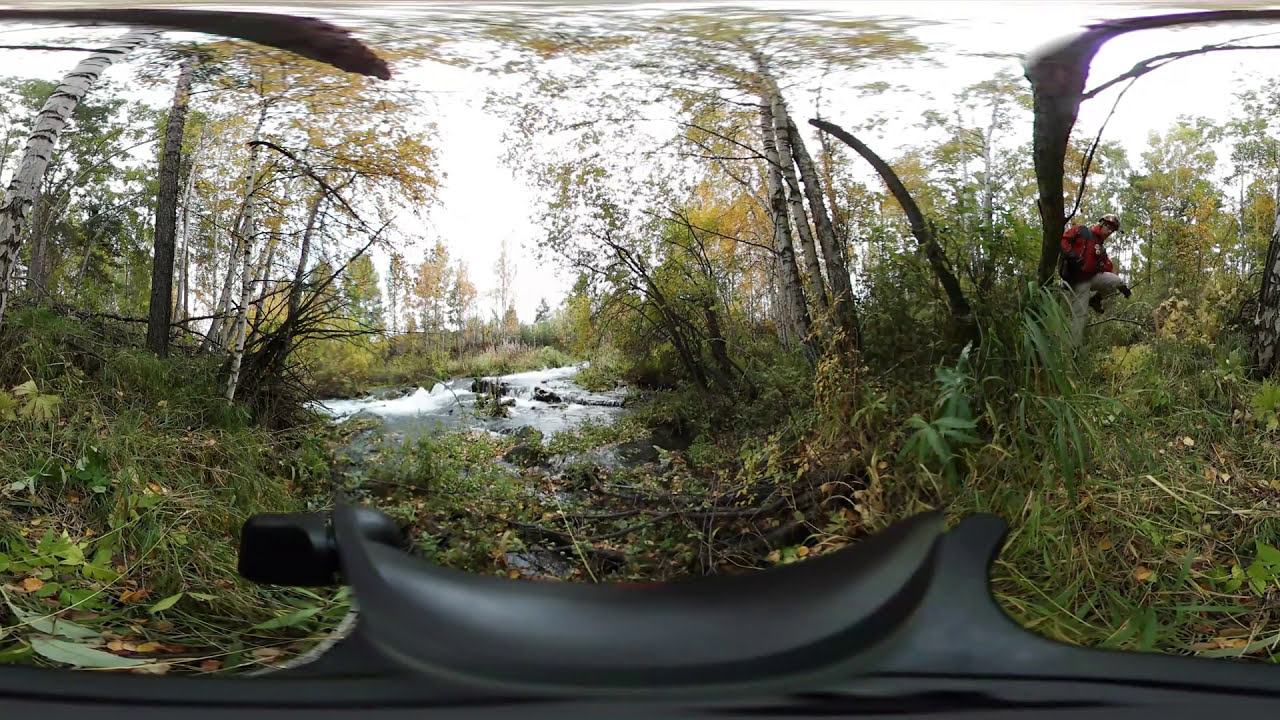The photo showcases a dense, marshy forest landscape with a wide, white-water river flowing through the center. The expansive scene is captured through a wide-lens or 360-degree panoramic shot, revealing three distinct sections. On the left, there are thick clusters of trees and grass. The central portion of the photo highlights the flowing river and marshlands, interspersed with a variety of flora, including grass, bushes, and leafless trees. The sky is visible, brightly lit, and peeking through the trees, emphasizing that the image is taken outdoors in broad daylight. Towards the right, a hiker clad in red and gray clothing with light tan pants, and a silver helmet is seen walking through the marshy area. The composition captures the vivid contrast of colors in the natural setting, featuring hues of green, brown, tan, white, yellow, orange, red, and highlighting the untouched beauty of the wilderness.